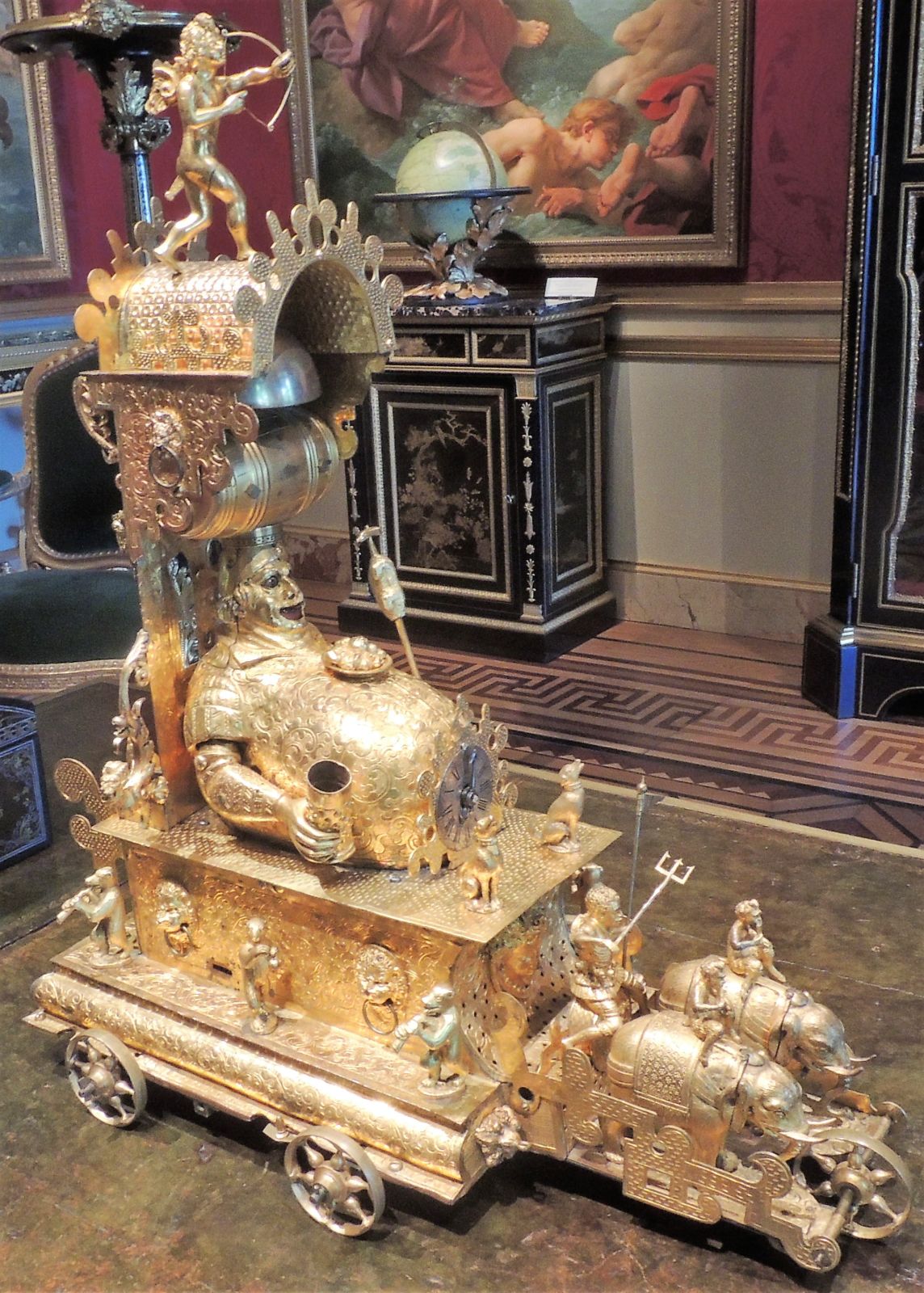The photograph, taken indoors—likely in a museum or a wealthy individual's home—features a highly detailed, golden metal sculpture that resembles an elaborate, ancient toy or collectible. This peculiar piece, slightly angled toward the bottom right, stands impressively large, almost five feet tall. At the base, two elephants, one ridden by a monkey, are positioned on a raised platform with a single wheel in the front. Above them, a man with a trident sits on an elevated seat.

The midsection of the sculpture showcases a notably rotund figure, larger than any other, whose legs are replaced by a clock. This figure reclines backward, with a plate of food on its belly and a golden cup in one hand, while the other hand remains hidden. Flanking this section, figures resembling bears or badgers appear to be playing musical instruments.

Crowning the sculpture is an arched structure, under which an angelic figure with a bow and arrow—a cupid—aims toward the right. Adding to the intricate craftsmanship, a small bell-topped instrument extends up and over behind the central rotund figure. The background of the photograph reveals red wallpaper on the upper half of the wall and light gray panels with gold trim on the lower half, along with some black Asian-style cabinetry.